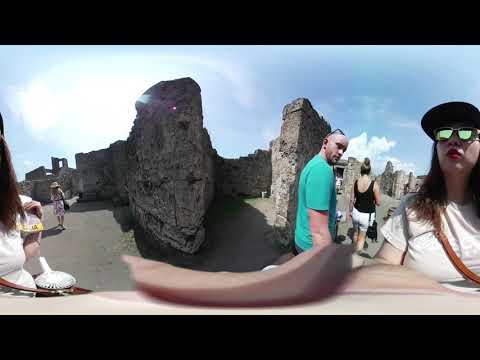The image depicts a panoramic view of a popular tourist site featuring ancient stone ruins, reminiscent of a castle or an old city with an Aztec or Machu Picchu-like vibe. The foreground showcases a stone path bordered by weathered stone walls, drawing the viewer's eye towards the depth of the scene. To the right, a woman with sunglasses, a baseball cap, and a white t-shirt stands prominently, her medium-length brown hair and red lipstick adding detail to her appearance. Her hand appears distorted due to the panoramic effect, looking elongated and squished.

Adjacent to her, a bald man sporting a lime-green (or teal) t-shirt and sunglasses perched on his head gazes back at her. Further down the path, more tourists can be seen, indicating the location's popularity. On the left side of the path, two women in summer dresses and hats stroll along, contributing to the bustling atmosphere. A person in a black tank top and white shorts is also visible, facing away from the camera.

The background reveals more of the ancient architectural ruins with walls of roughly hewn stones forming tight enclosures and rooms. The sky overhead is blue with sporadic clouds dotting the expanse. The scene is both vibrant and historic, capturing a moment where modern visitors explore time-honored remnants of a distant past.